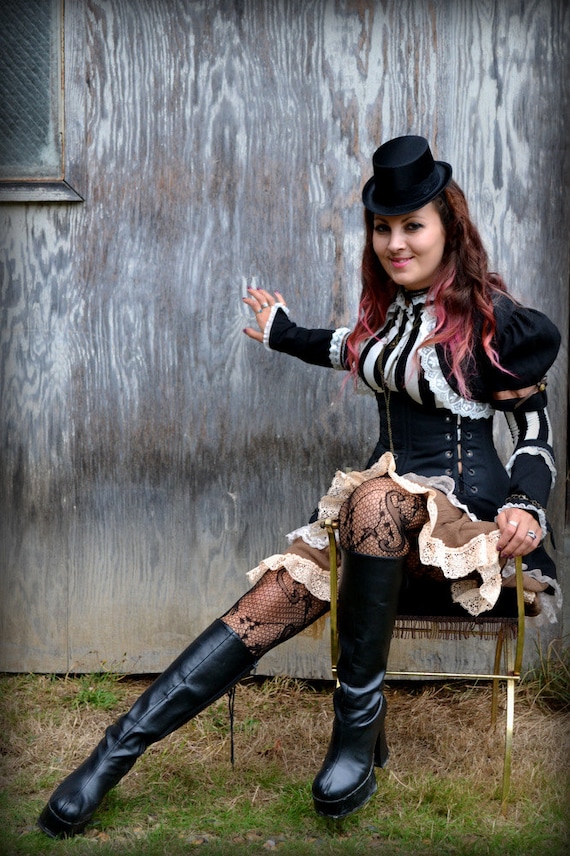This image captures a woman dressed in an elaborate, Victorian-inspired costume, characterized by a black and white color palette. She's seated on a small brass stool on grass that appears somewhat brown and dying, in front of a grayish wooden wall with a window in the upper left corner. Her outfit consists of a black leather corset with visible strings around her waist area, puffy black sleeves adorned with white lace, and black and white striped top. She wears thigh-high, shiny black leather boots, possibly paired with fishnet stockings, and sports a small black top hat. Her long brown hair has distinct red or pink highlights. She is accessorized with several silver rings on both hands, with a smile on her face and reaching out with one hand. The setting suggests a rustic, possibly worn-down environment, adding to the overall vintage and somewhat whimsical aesthetic of the scene.